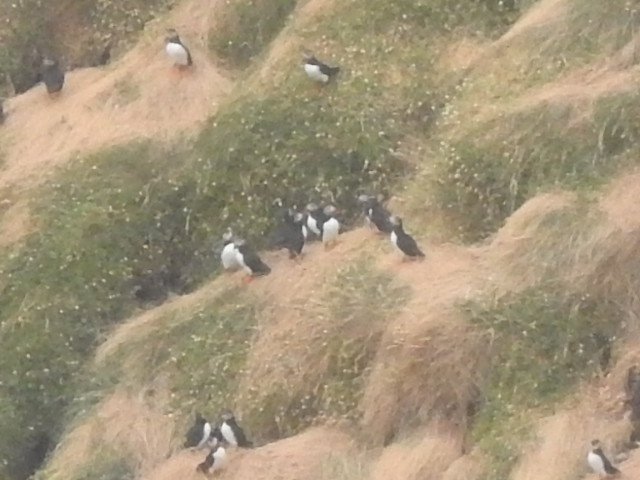The image is an outdoor, low-quality, slightly blurred color photograph, capturing a steep, undulating hillside that ascends to the right away from the camera. The hillside is characterized by a mix of long, light brown, yellowish straw and patches of green grasses that feature scattered lines and specks of white, likely wildflowers or weeds. Throughout the hillside, random clusters of birds, which bear a resemblance to penguins or possibly auks, are seen. Due to the low image quality, the exact species of the birds cannot be determined, but they are notable for their distinct black and white coloring: white breastplates and bellies with dark black feathers on their heads and backs extending to their tails. Some birds in the middle of the image appear to have light brown or orange feet. The birds are dispersed across the hill, with more concentrated groups observed towards the middle and lower sections of the hillside.